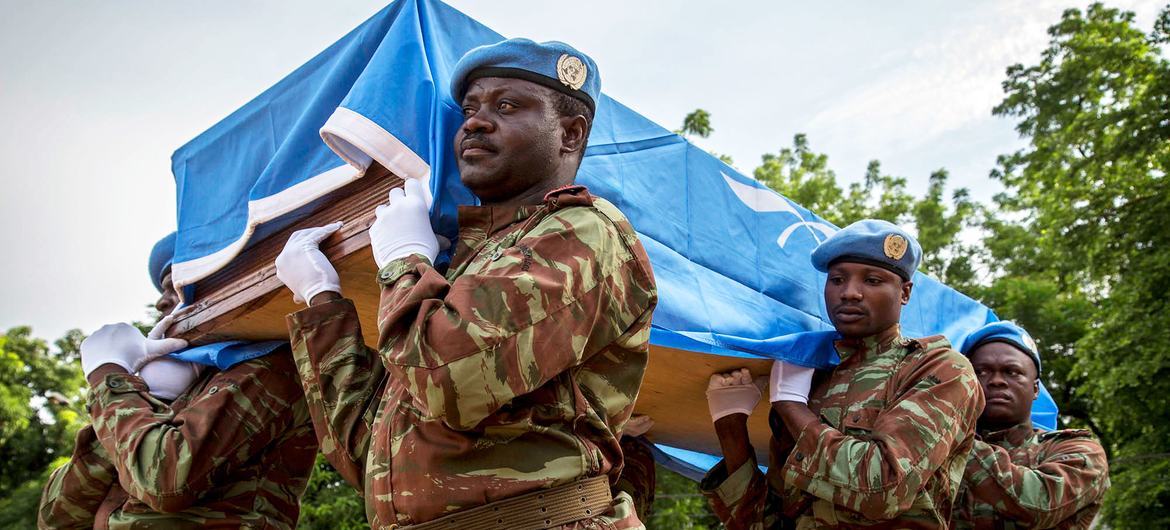In this outdoor image, a solemn group of soldiers is carrying a wooden casket draped with a blue cloth in a likely military funeral. The bearers, dressed in camouflage uniforms, wear blue berets adorned with gold emblems, possibly signifying their affiliation to an international organization like the United Nations. There are at least six men carrying the casket—three clearly visible on the left side facing the camera, one in the front on the right, and at least two others implied. Their serious expressions and averted gazes underscore the gravity of the moment. The background features green trees and a sky that transitions from light blue to white clouds, suggesting a peaceful setting, possibly in a country like Mali or Uganda.